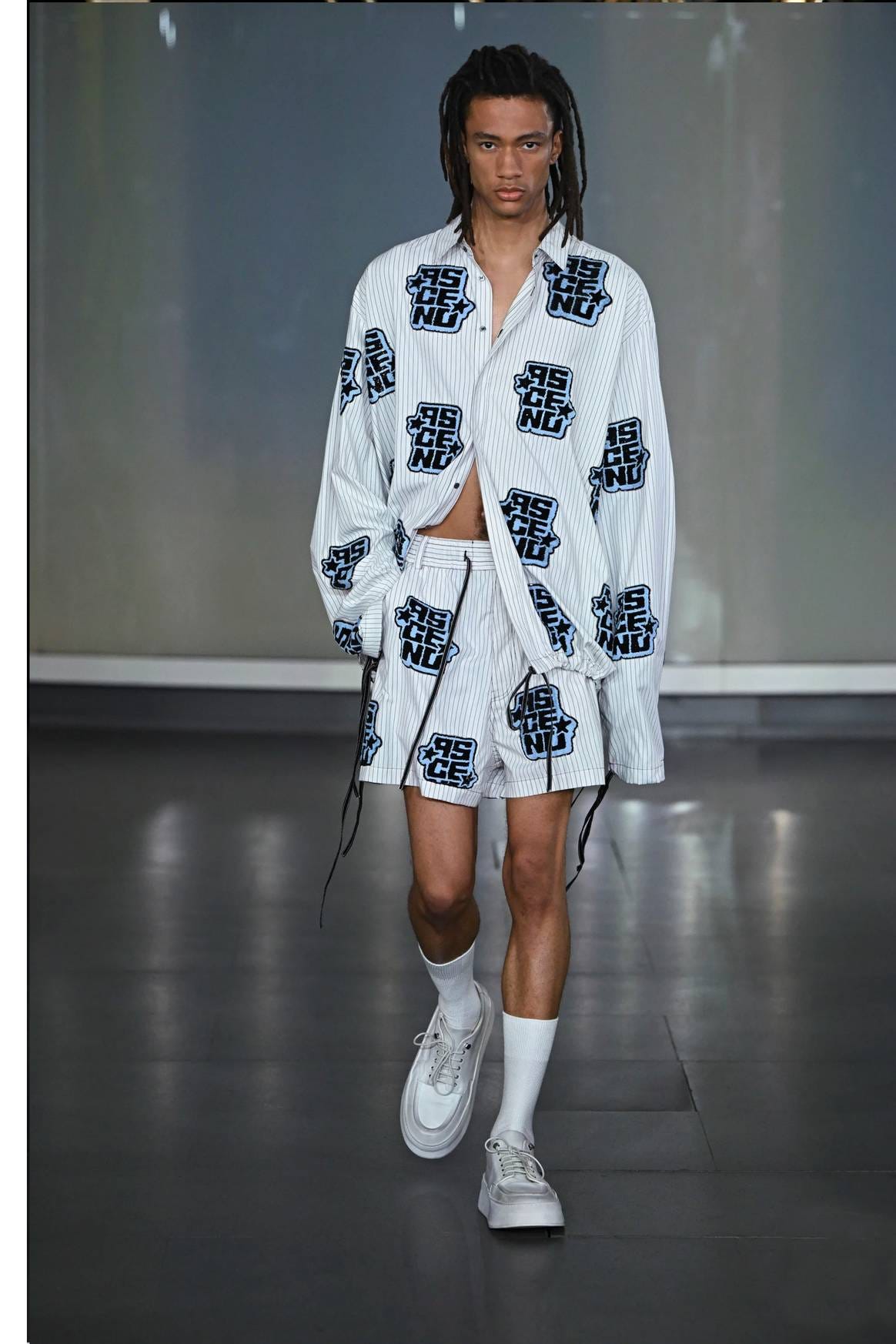The image captures a male model with dark skin and dreadlocks, walking indoors on a dark gray runway, set against a gray wall that may serve as a stage backdrop. The model is wearing a coordinated outfit consisting of a long-sleeve, collared white shirt and matching white shorts. The shirt, which is not fully buttoned, features small black and white patches that spell out "ASCEND" vertically with the breakdown of letters reading "AS" on one line, "CE" on the next, and "ND" on the bottom line. These patches, containing the letters A-S-C-E-N-D and two stars on either side, are scattered uniformly over both the shirt and shorts. The ensemble is completed with white socks pulled up to the calf and white tennis shoes. The model's right hand is in his pocket while his left hand remains unseen, and he appears to be walking with his gaze fixed directly ahead, possibly at the camera, capturing him in mid-motion on the runway. The image's indoor setting is illuminated by overhead lighting, casting a bright ambiance that highlights the cleanliness and minimalism of the scene.